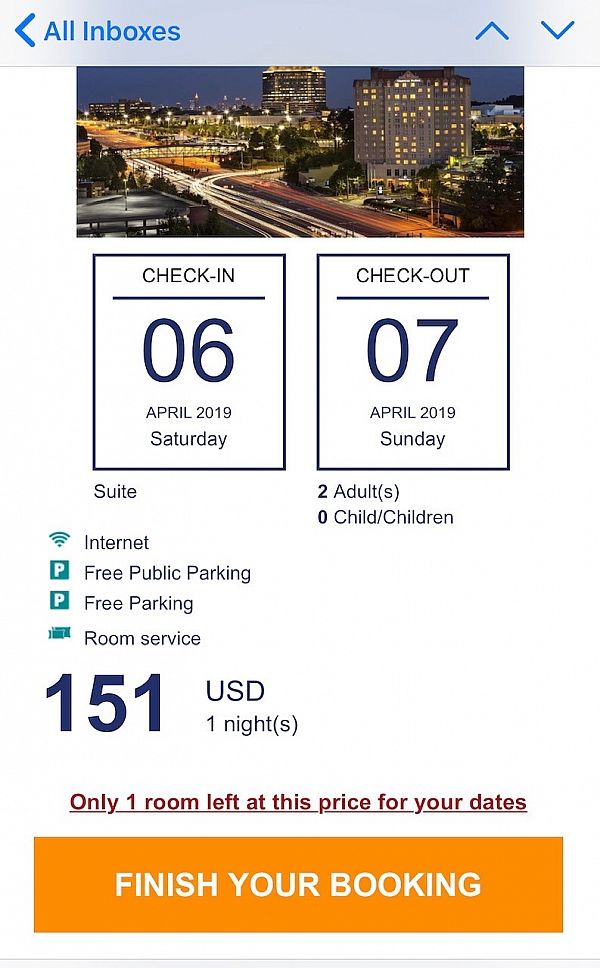The image features a vibrant ombre background transitioning from white at the top to a bluish hue towards the bottom. On the left side of the image, there is a blue arrow pointing left. The top right corner displays two arrows, one pointing up and the other pointing down. Below this, there is a dark scene depicting a silhouetted cityscape with towering buildings illuminated by gray lights along a road. 

The middle section features a white background with two detailed blue boxes. The left box, colored in dark blue, contains the text "Check In," followed by a horizontal line underneath with the date "06 April 2019, Saturday." The right box is similarly formatted, stating "Check Out" with a line underneath detailing the date "07 April 2019, Sunday." Below these boxes, the left side reads "Suite," while the right side states "Two adults," with "(S)" in parentheses and "0 child/children" below it.

The bottom section lists several amenities in blue text: "Internet, Free public parking, Free parking, Room service." Beneath this, the price is specified as "$151 USD" for "1 night(s)." In red, underlined text, it warns, "Only one room left at this price for your dates." 

An orange box at the bottom of the image with bold white capital letters encourages the viewer to "FINISH YOUR BOOKING," indicating that the user is at the final step of reserving the room.